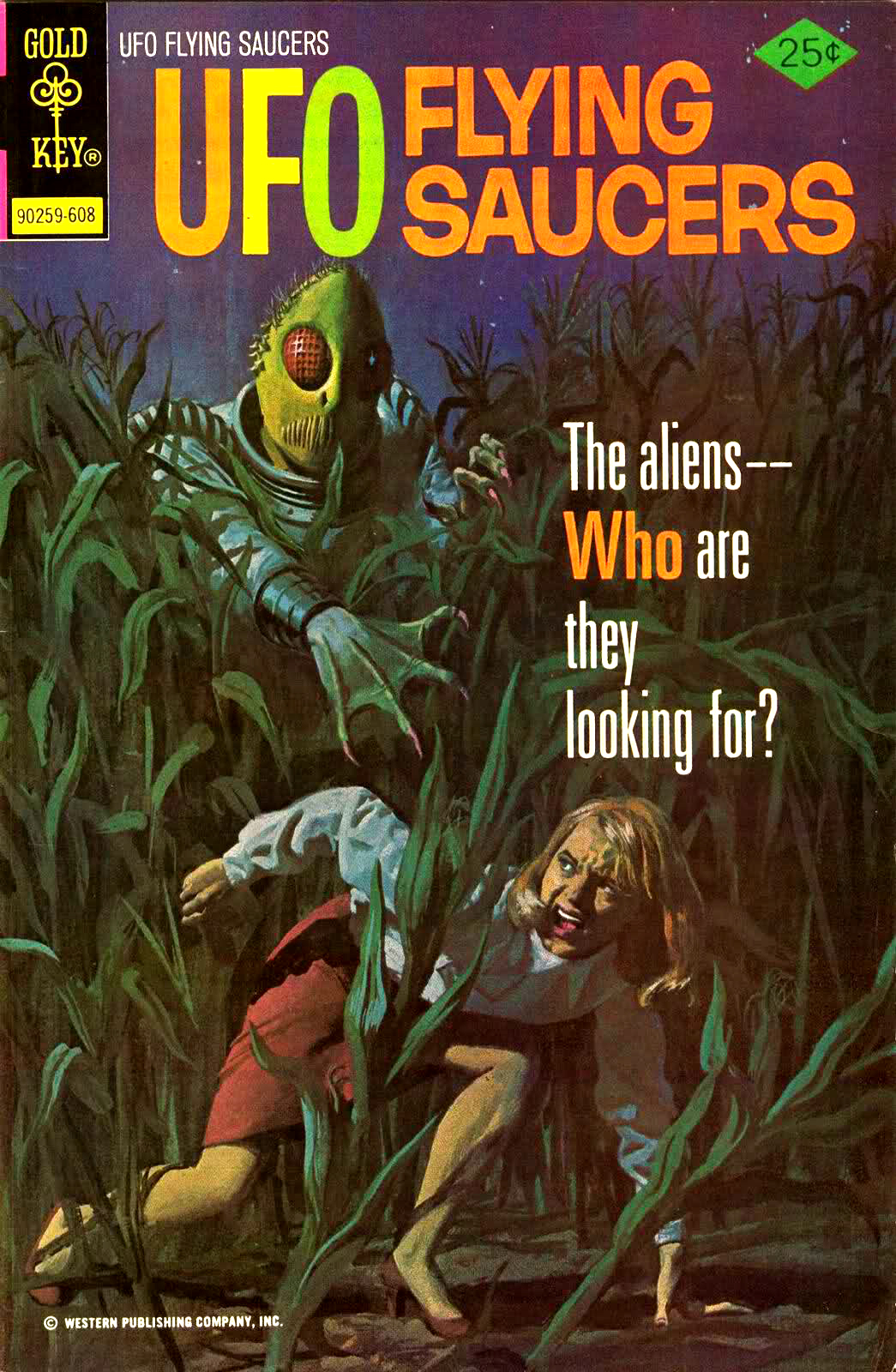The cover of this vintage magazine, titled "UFO Flying Saucers," features a chilling scene set in a cornfield. In the top left corner, there's a Gold Key logo, accompanied by the numbers 90259-608, while the upper right corner displays a green diamond indicating the price of 25 cents. The title "UFO Flying Saucers" appears prominently in white letters at the top, with additional text below asking, "The aliens. Who are they looking for?" 

The central image depicts a terrifying encounter between a young woman and a classic reptilian alien. The alien, characterized by its green head, red insect-like eyes, and webbed hands, wears a space suit as it emerges from the cornfield, reaching toward the woman. She is a blonde with shoulder-length hair, donned in a light blue or white blouse and a red skirt that falls just above her knees. The scene captures her mid-flight, fear evident as she stumbles in her attempt to escape the alien's grasp. At the bottom of the cover, there's small text that reads, "Copyright Western Publishing Company Incorporated."